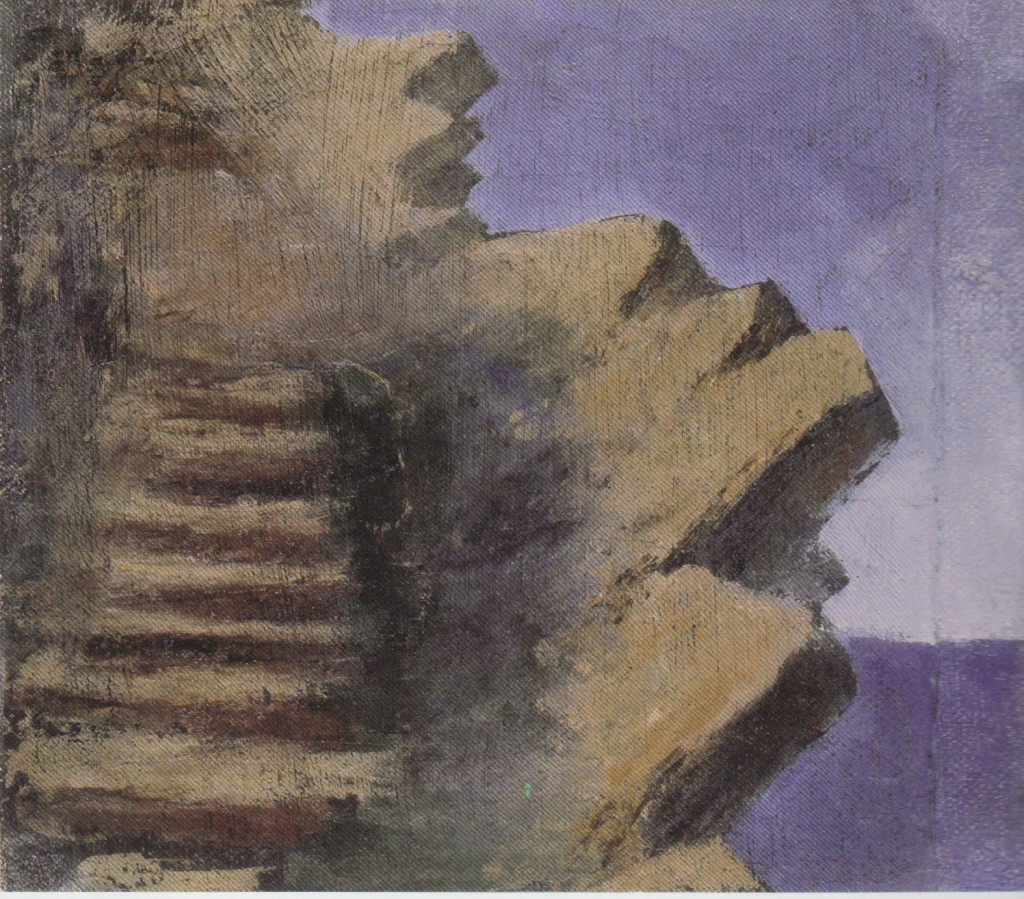The painting portrays a jagged rock cliff with a stone stairwell that ascends its rugged side, overlooking a vast ocean. The cliff juts out with sharp, jagged edges in hues of brown, dark brown, black, and gray, resembling the teeth of a zipper. The stairwell, comprised of varying stair sizes, winds its way up the left side of the cliff, starting with a small step and progressing to larger ones, and finally narrowing at the top, forming a subtle 'S' shape. The right side of the stairs is enveloped in black shadows, contrasting with the light brown path above. Below, a patch of blue ocean is visible, suggesting the height and precariousness of the stairwell. The sky above transitions from ominous purples and stormy clouds to a lighter, faded center at the horizon, enhancing the dramatic and moody atmosphere of the scene. The overall color palette is muted and earth-toned, contributing to the painting's subtle, realistic yet not overly detailed style.